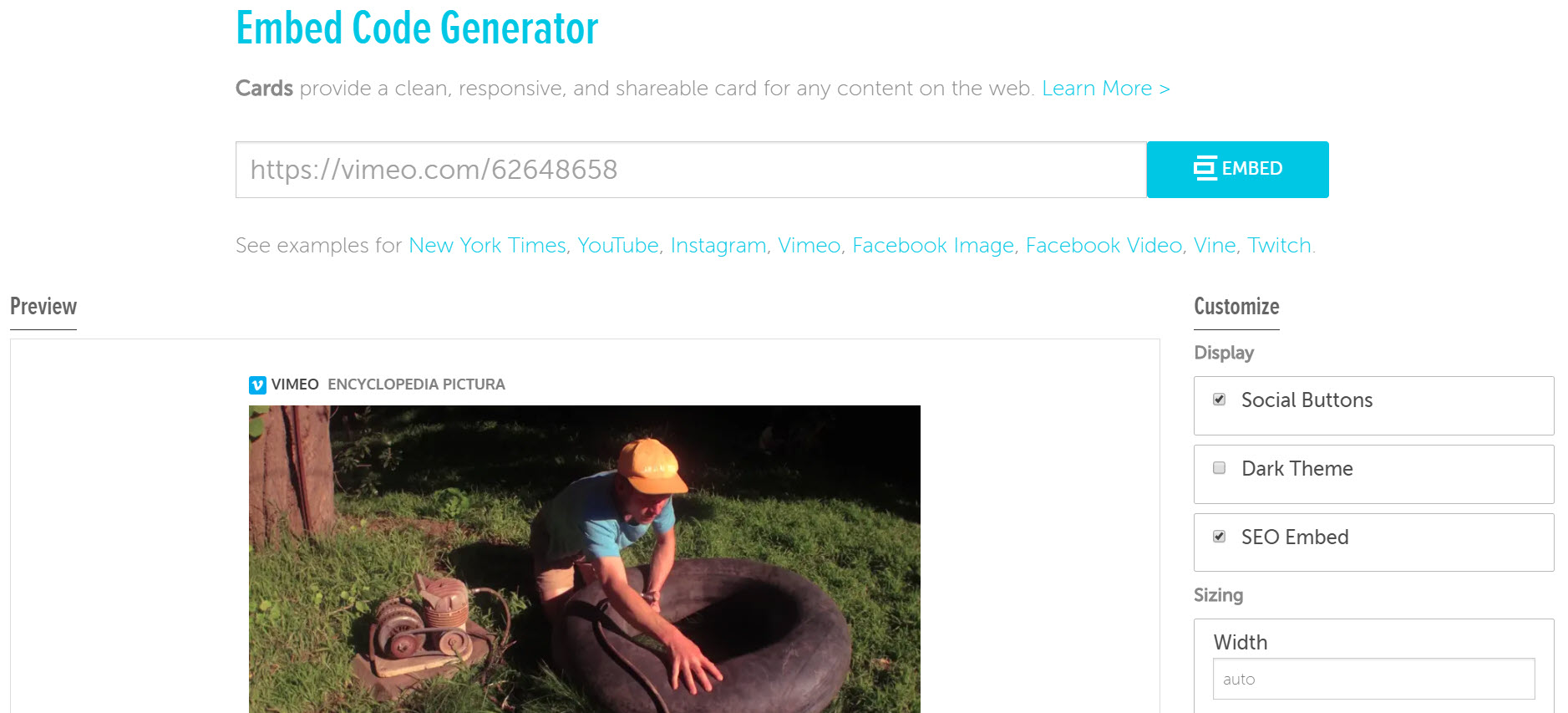The image depicts a website interface designed to generate embed codes for videos. The background is predominantly white, and in the top-left corner, the header reads "Embed Code Generator" in light blue. Below this, a gray subheader states, "Cards provide a clean, responsive, and shareable card for any content on the web." To the right of this subheader, "Learn more" appears in light blue with a right-facing arrow. 

The word "Cards" at the beginning of the subheader is in bold. Directly below, there is a white text input box with the placeholder "https://vimeo.com/". Accompanying this box is a blue "Embed" button to its right. Further down, a line of text lists examples of content sources: "New York Times, YouTube, Instagram, Vimeo, Facebook Image, Facebook Video, Vine, Twitch."

To the left below this text, there is a label "Preview." Centrally, there is a preview thumbnail featuring an image from Vimeo. The thumbnail shows a man inflating a tire, donning a blue shirt and an orange hat. Above this thumbnail, the text "Vimeo Encyclopedia Pictora" is displayed. 

On the right-hand side of the interface, a series of configuration menus are visible. These include options such as "Customize" and "Display," with the "Social buttons" toggle marked as checked. "Dark theme" remains unchecked, while "SEO Embed" is checked. Below these options, a field labeled "Width" contains an empty text box. The image of the man inflating a tire is centrally framed, embodying the function of the embed code generator to incorporate such visual content seamlessly.